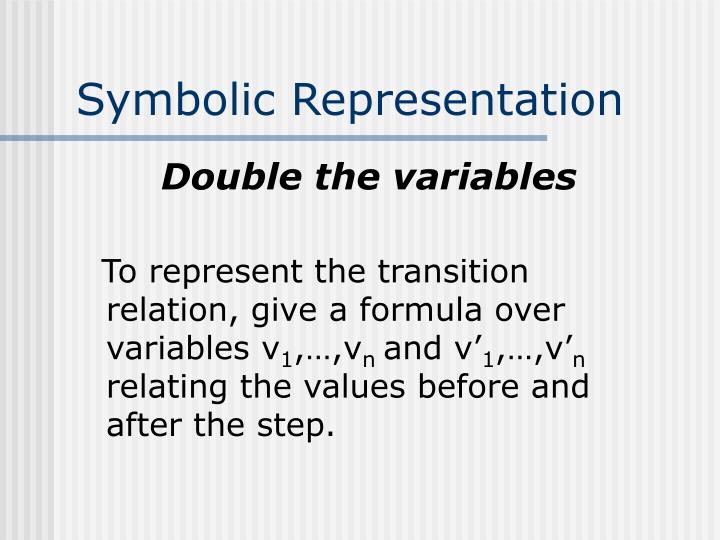This image appears to be extracted from a Microsoft PowerPoint presentation slide. The background features vertical, alternating gray and transparent white stripes, except for a darker gray section on the far left. Dominating the top portion of the slide is the title "Symbolic Representation," written in blue font, accompanied by a horizontal blue line immediately below it. Directly beneath this line, the text "Double the variables" is prominently displayed in bold, black font. Further down, an explanatory note in black font reads: "To represent the transition relation, give a formula over variables v1, ..., vn and v'1, ..., v'n relating the values before and after the step." The entire slide conveys detailed instructions on doubling variables and appears as part of a structured slideshow presentation.